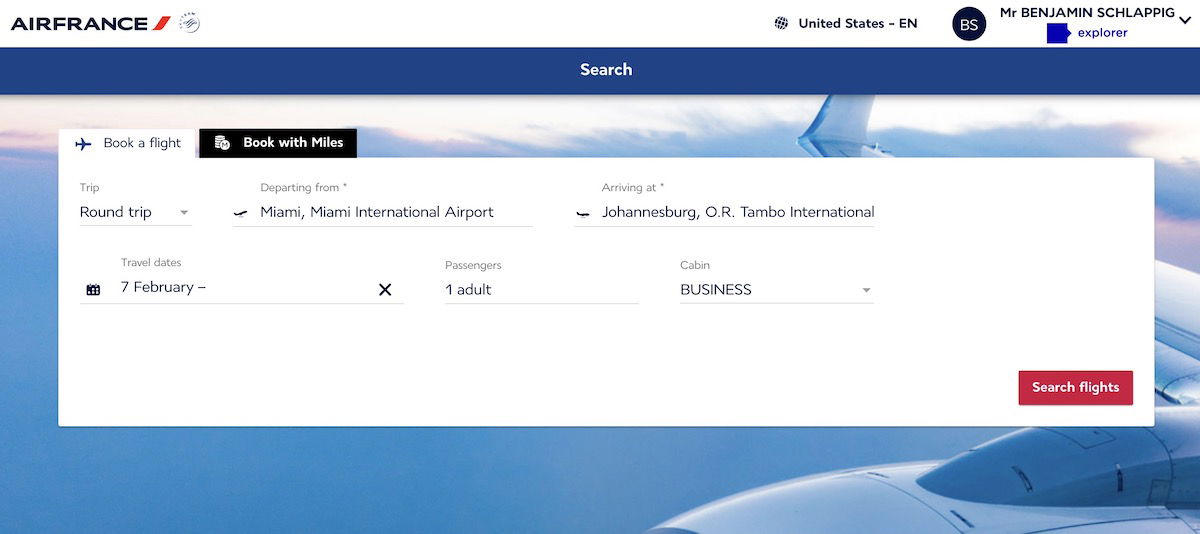The image displays a detailed interface of an Air France flight booking webpage. Located at the top left is the "Air France" logo followed by a small red icon. To the right along the top bar, it reads "United States-EN." Adjacent to this, a small black circle contains the initials "BS" next to the text "Mr. Benjamin Schlappig." Below this, a blue button labeled "Explore" is present.

A wide blue bar beneath these elements features a "Search" label. Below the bar, there is a cropped image of an airplane in the sky, only partially visible. Central to the interface is a large white box containing several tabs; the top tabs are labeled "Book a Flight" and "Book with Miles."

Within the white box, several information fields have been filled in. The "Trip" section specifies a "Round Trip," departing from "Miami, Miami International Airport," and arriving at "Johannesburg OR Tambo International." The "Travel Dates" section lists "7 February" with an unspecified return date, indicated by a dash. The "Passengers" field states "One Adult," and the "Cabin" indicates "Business Class."

In the bottom right corner of this section, a prominent red button labeled "Search Flights" invites users to initiate their flight search.